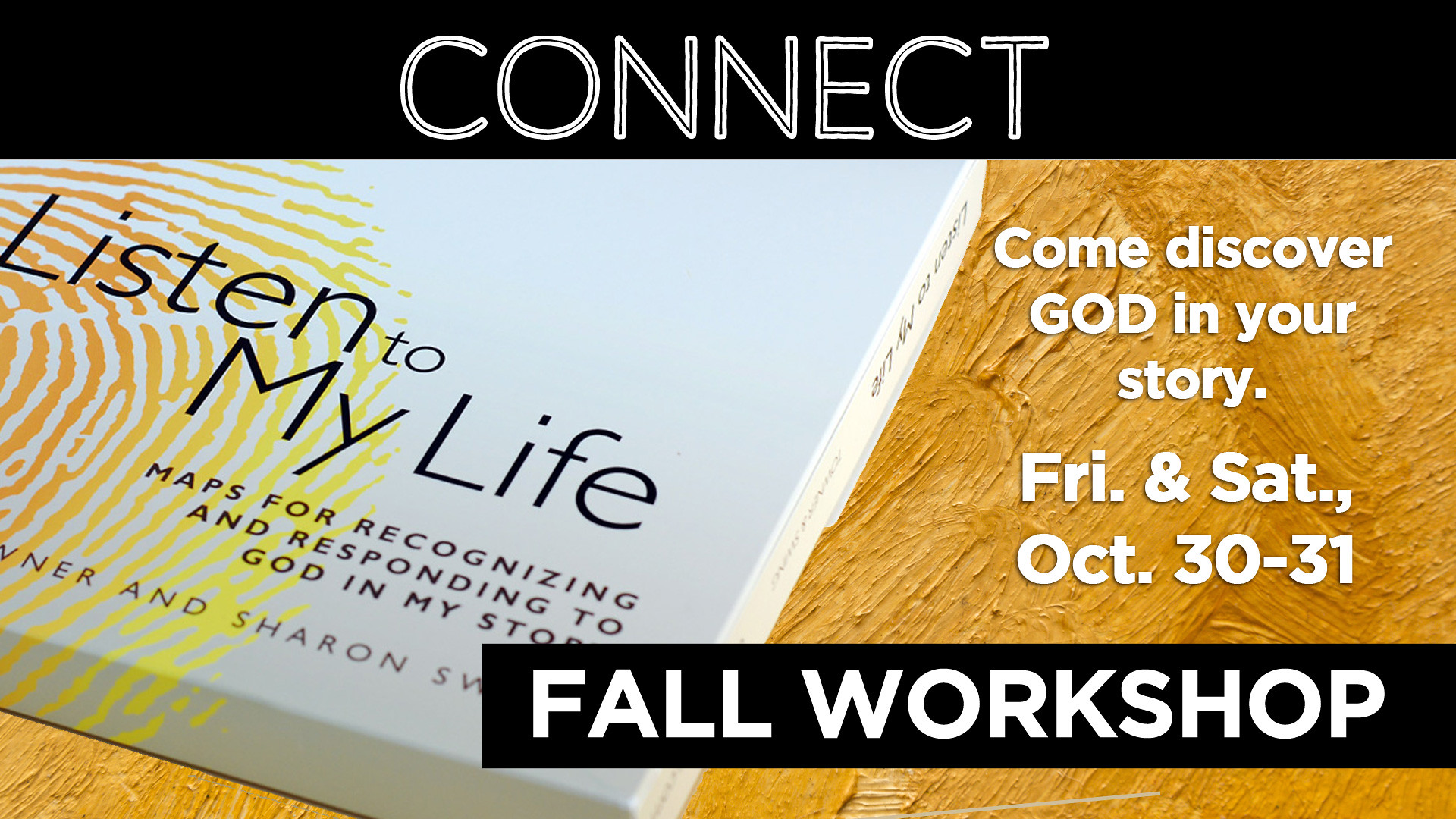The image is an advertisement for a "Fall Workshop," prominently featuring a black banner at the top with the word "CONNECT" in large white capital letters. Below this banner, to the left, there's a white rectangular box, possibly a book, placed on a wooden table. The book's cover displays an orange and yellow fingerprint design and bears the title "LISTEN TO MY LIFE" in black text. Beneath the title, the tagline reads "Maps for Recognizing and Responding to God in My Story," although part of the text and the authors' names are partially cut off, revealing only "Weiner" and "Sharon Sv." To the right side of the image, in white text, it invites viewers to "Come discover God in your story," specifying the event will take place on Friday and Saturday, October 30th to 31st. At the bottom, another black banner with "FALL WORKSHOP" in white capital letters completes the announcement.